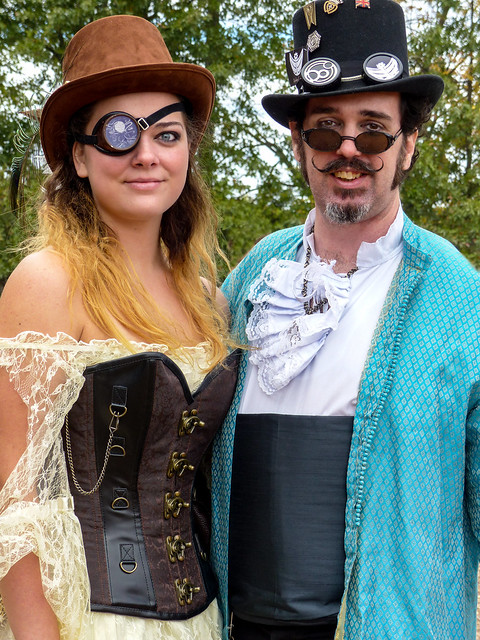The photograph captures a steampunk-themed duo set against a backdrop of trees and a blue and white sky. On the right stands a man, adorned in a black top hat decorated with steampunk goggles and various pins. His facial features include brown sideburns, a curly-tipped mustache, a goatee, and a whimsical smile that reveals three yellow teeth. He is dressed in a white ruffled shirt beneath a blue jacket and a black vest. On the left is a woman with a brown velvet top hat, her long wavy hair transitioning from blonde to light brown. She sports a monocle goggle over her right eye and wears a lacy off-the-shoulder bustier that forms part of a light yellow dress. Her ensemble is completed with a corset-style vest adorned with a chain. Both individuals embody the intricate and distinctive aesthetics of steampunk fashion.